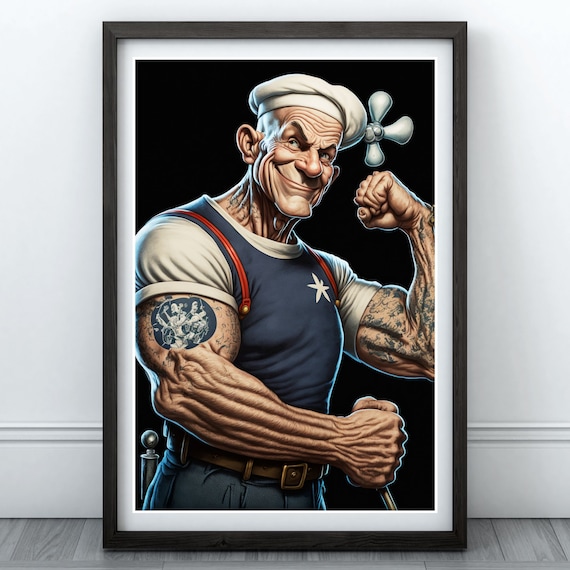This framed poster leans against a white wall on a gray floorboard. Captured within a dark gray frame with a white lining, the image is a digital, photorealistic caricature reminiscent of Popeye the Sailor Man. The character sports a white hat with a peculiar faucet handle-like propeller on one side, paired with big ears and a broad smile. His wrinkled face and neck complement his exaggerated muscular physique. He's flexing with fists clenched, showcasing rippling muscles and popping veins on his forearms and upper arms, which are heavily tattooed. Dressed in a blue shirt with white sleeves and a star above the left breast, along with a belt and blue pants, the figure’s attire completes the modern yet nostalgic depiction.